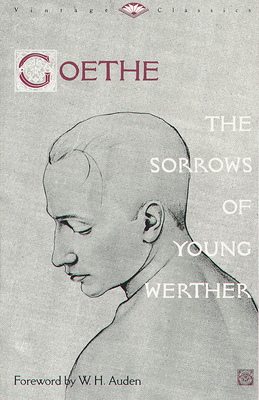The image is a detailed depiction of a book cover with a vertical rectangular layout on a gray background. At the top, in black text, it reads "Vintage Classics," with a small insignia centered between the two words. Below this title, in bold red letters, the name "GOETHE" is prominently displayed, where each letter is enclosed within a light gray square. Underneath the author's name, there is a stylized, black-and-white silhouette drawing of a man with his head turned slightly downward to the left, capturing his upper body and neck, with a hint of sadness in his posture.

To the right of this illustration, in white text, the book's title "The Sorrows of Young Werther" runs vertically from the man's head down to his shoulders. At the bottom left corner of the cover, there is a smaller black text indicating "Foreword by W.H. Auden." Adjacent to this, in the bottom right corner, a small red square insignia is also present. The overall theme of the cover is monochromatic with red accents, contributing to the somber and reflective tone conveyed by the illustration of the man.